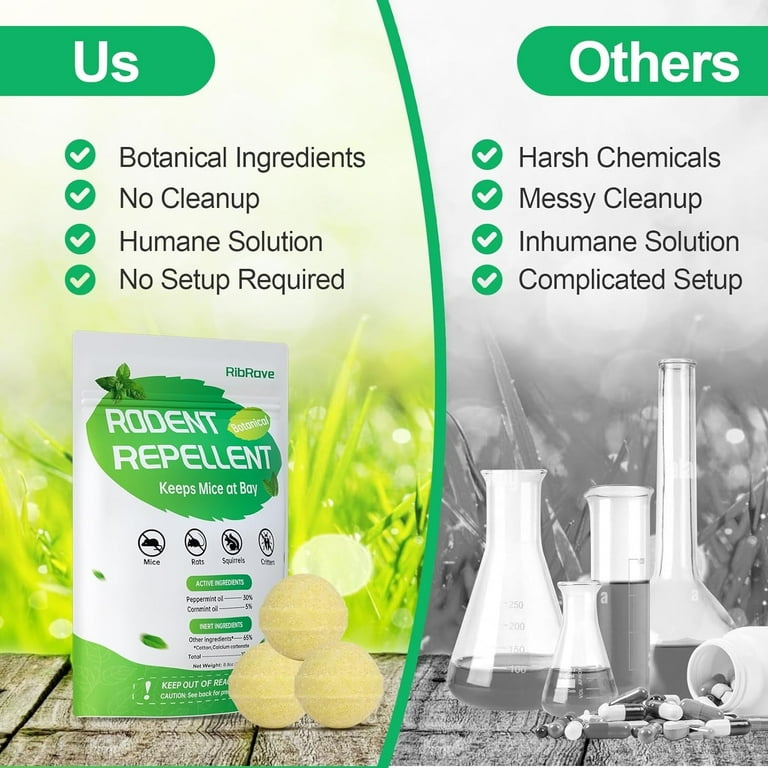This advertisement for Rib Rave's Rodent Repellent features a compelling side-by-side comparison with its competitors. The image is split vertically by a green line; the left side, labeled "US," has a green hue, while the right side, labeled "Others," is in black and white. On the left, a green box prominently displays "US," followed by four green check marks next to the benefits: "Botanical Ingredients," "No Cleanup," "Humane Solution," and "No Setup Required." Below this, the Rib Rave Rodent Repellent product is showcased on a wooden deck. The product is in a white bag with a large green leaf and the text "Rodent Repellent - Keeps Mice at Bay," accompanied by a safety warning to keep away from children. The bag is surrounded by three yellowish eggs and framed by green grass in the background.

On the contrasting right side, labeled "Others," four negatives are listed with black X marks: "Harsh Chemicals," "Messy Cleanup," "Inhumane Solution," and "Complicated Setup." This section depicts test tubes and pills arranged on a wooden deck, with a grainy black-and-white grassy background, emphasizing a less favorable approach. The advertisement strongly advocates for Rib Rave's humane and hassle-free product over traditional, chemical-based solutions.